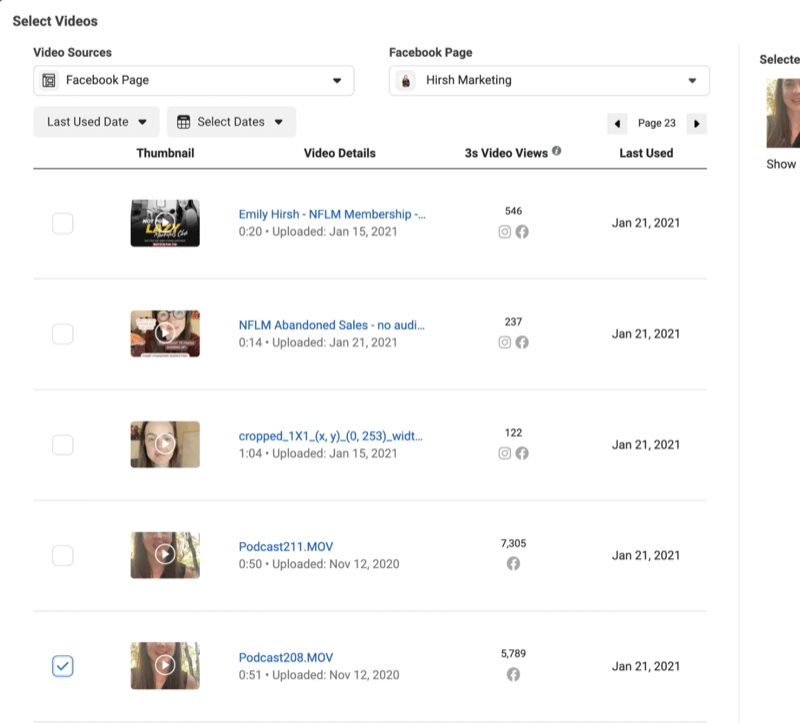The image depicts a user interface with a predominantly white background, outlined in light blue. At the very top, a header labeled "Select Videos" is displayed. Below this, there's a section labeled "Video Sources," containing a dropdown box with an inner black rectangle labeled "Facebook Page," accompanied by a downward arrow. The dropdown box is repeated, also labeled "Facebook Page," and features a smaller gray box with a brown icon reading "Hirsch Marketing," also with a downward arrow.

Underneath this, there's a button labeled "Last Used Date" with a downward arrow and another dropdown labeled "Select Dates" with a downward arrow. Adjacent to these, navigation controls include a box with a left arrow labeled "Page 23" and a blue box with a right arrow.

The main content area is structured in several columns titled "Thumbnail," "Video Details," "3s Video Views," and "Last Used," with a small gray circle featuring an "I" symbol. A prominent gray line divides this section. 

Several entries are listed:

1. An empty selection box next to the first entry featuring a thumbnail image, labeled "Emily Hirsch NFL Membership," uploaded on January 15, 2021, at 5:46. It includes a small square icon and a Facebook timestamp of January 20, 2021.
2. Another entry labeled "NFL M Abandoned Sales," uploaded on January 21, 2021, at 2:37, with corresponding Facebook timestamp on the same date. 
3. A cropped image of a girl with details of the video upload and Facebook timestamp repeated below.
4. A video titled "Podcast 211.mov," uploaded on November 12, 2020, at 7:05, with a Facebook timestamp of January 21, 2021.
5. The final entry, labeled "Podcast 208.mov," includes a blue-checkmarked selection box, a thumbnail image of a girl, and the upload timestamp along with the Facebook date of January 21, 2021.

A light blue line runs down the side of the interface, and in the upper right corner, there is a profile image of a girl accompanied by the label "Show."